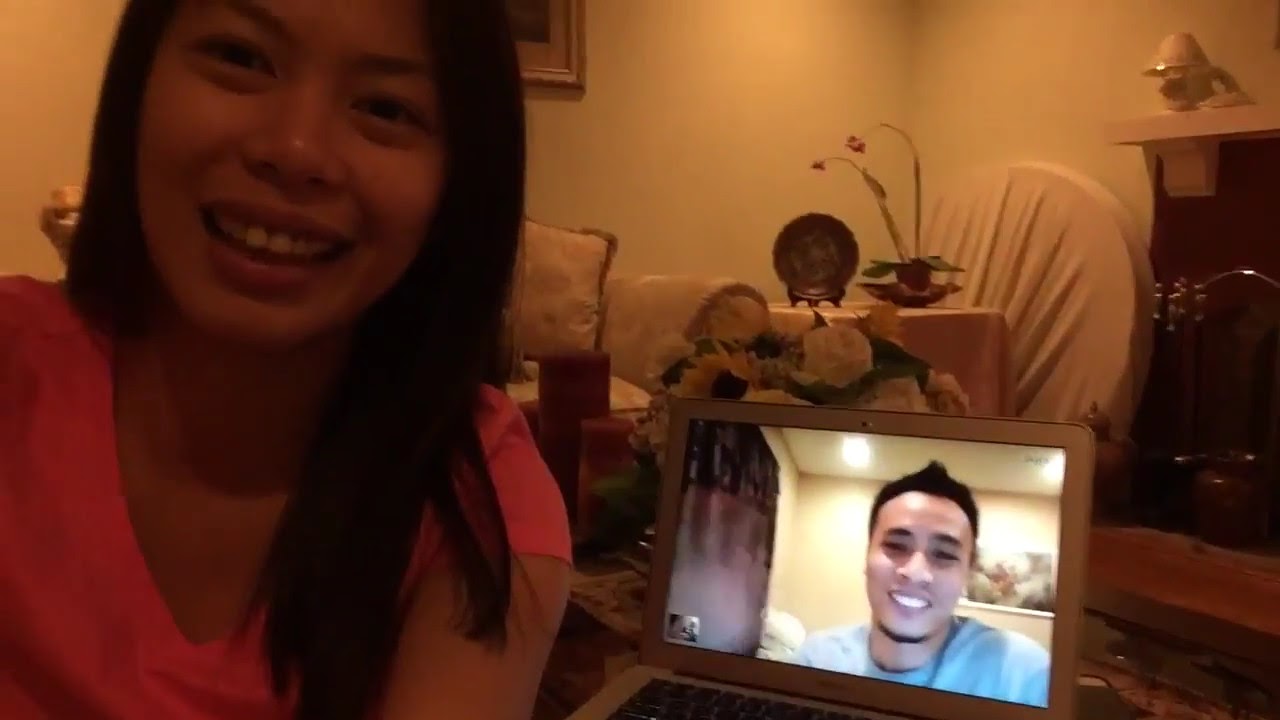In this image, a close-up of an Asian woman occupies the left side, where she is seen from the chest up, wearing a pinkish-orange v-neck t-shirt, with long, dark shoulder-length hair, and is smiling directly at the camera. To her right is an open laptop, likely an Apple device, displaying a live video chat such as FaceTime or Zoom. On the laptop screen, a young man with darker skin, a small black goatee, short spiky black hair, and a bright smile is visible, wearing a blue shirt. The setting appears to be a comfortably furnished residential room with beige walls and soft, dim lighting. Behind the woman, there is a cushioned couch, a vase of flowers, red candles, and some covered furniture, including a table with decorative items like a plate and some orchids. Additionally, the image captures a glimpse of a fireplace and mantle on the far right, adding to the cozy and welcoming atmosphere.